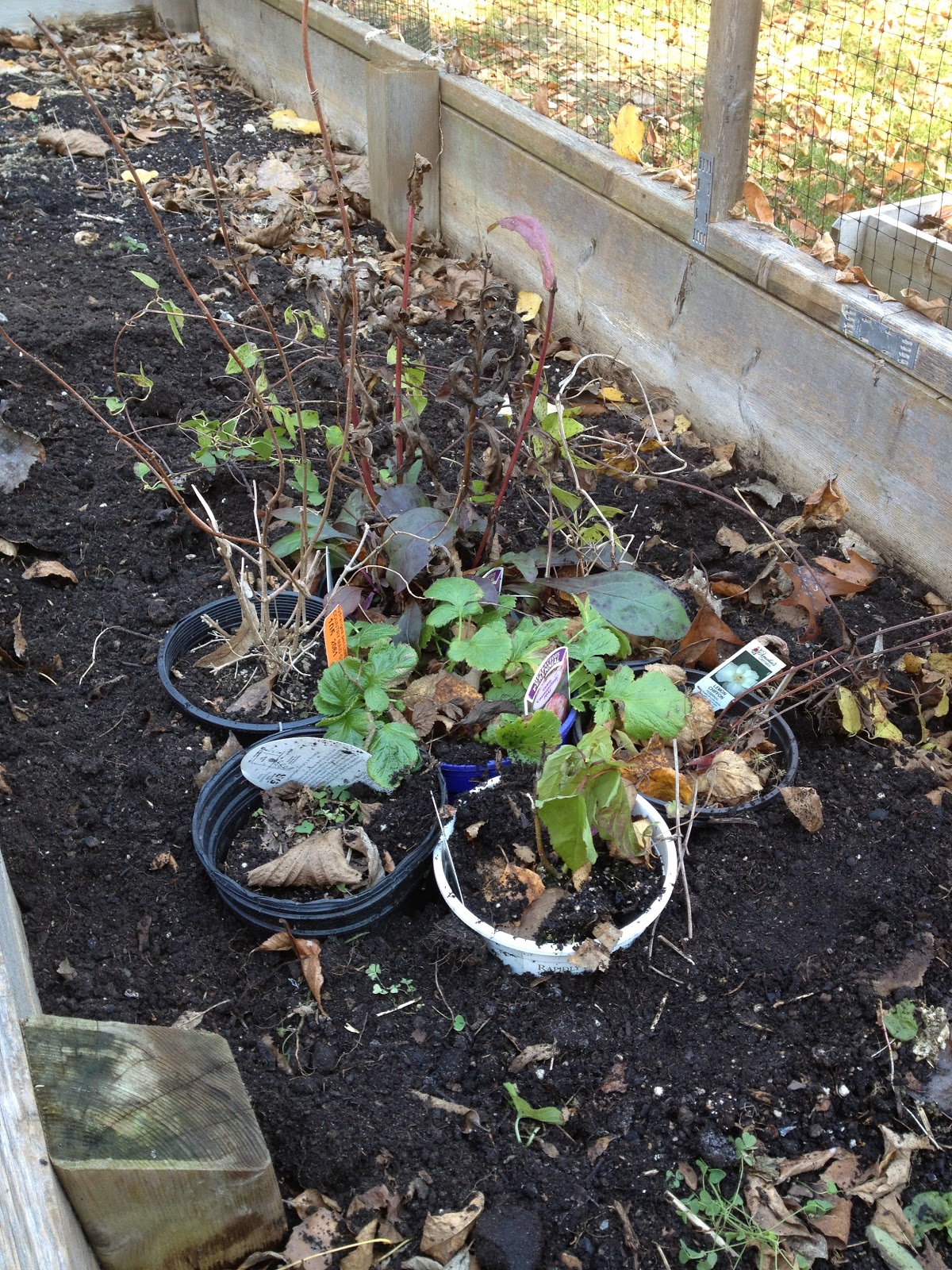This is a vertically-oriented color photograph capturing a fall garden scene. The garden bed, enclosed by a wooden and metal frame, features rich, dark brown, loamy soil that appears exceptionally fertile. The most prominent elements in the image are four potted plants arranged in the center, their pots varying in color from white to black to dark blue. These pots are closely positioned, touching each other, and several have plastic descriptive photos and labels still attached.

The plants in the pots exhibit a mix of life stages. Some of the taller stalks have dried leaves or are entirely barren, while the surrounding plants still retain a few green leaves amidst the dried and dying foliage, indicating the transition into fall. The garden bed also has scattered dried brown leaves, adding to the seasonal atmosphere.

The garden is partially protected by a mesh fence at the top right corner, designed to keep out pests and animals. This wire fencing is supported by wooden stakes and extends around the perimeter of the garden. Beyond the mesh fence, a vibrant green lawn sparkles under the sunny light, providing a contrasting backdrop to the subdued colors of the fall garden. Additionally, there is a wooden fence post at the lower left-hand corner, further defining the garden's boundary. Overall, the scene conveys a sense of potential and readiness, despite the seasonal decay.